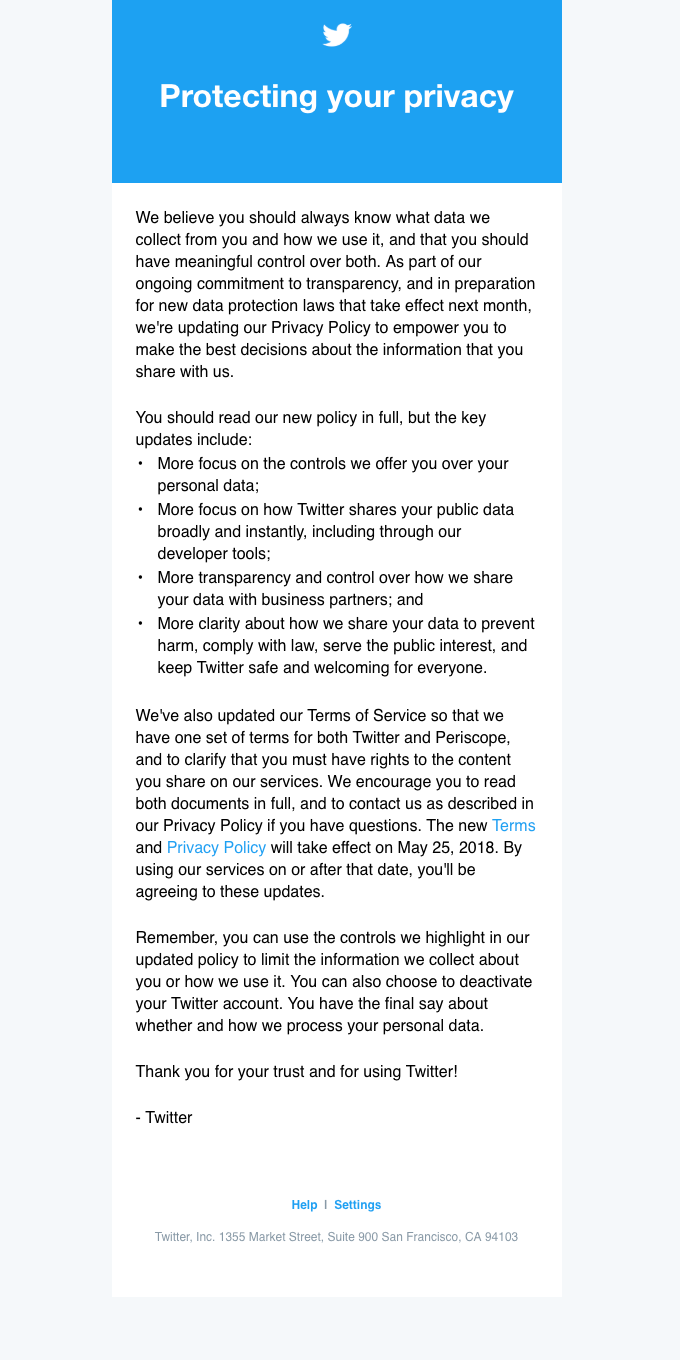The image depicts a screenshot from a website with a light gray background. Prominently positioned at the top center is a medium blue banner featuring the Twitter (now X) logo, a blue bird. Beneath the logo, in bold, it states, "Protecting Your Privacy," with "Protecting" capitalized.

Below the banner, against a white background, there is detailed text about Twitter's privacy policy updates. The message emphasizes Twitter’s commitment to transparency, highlighting that users should always be informed about the data collected and how it's used. The text explains that the company is updating its privacy policy in preparation for new data protection laws coming into effect next month. 

The update aims to give users more control over their personal data, focusing on several key areas:
1. Enhanced controls over personal data.
2. Greater transparency concerning the sharing of public data, especially through developer tools.
3. Improved clarity on data sharing with business partners.
4. More explicit guidelines on data sharing for preventing harm, complying with legal requirements, setting public interest, and maintaining a safe environment on Twitter.

The message encourages users to read the new policy in its entirety and concludes with a note of gratitude for users' trust and continued use of Twitter.